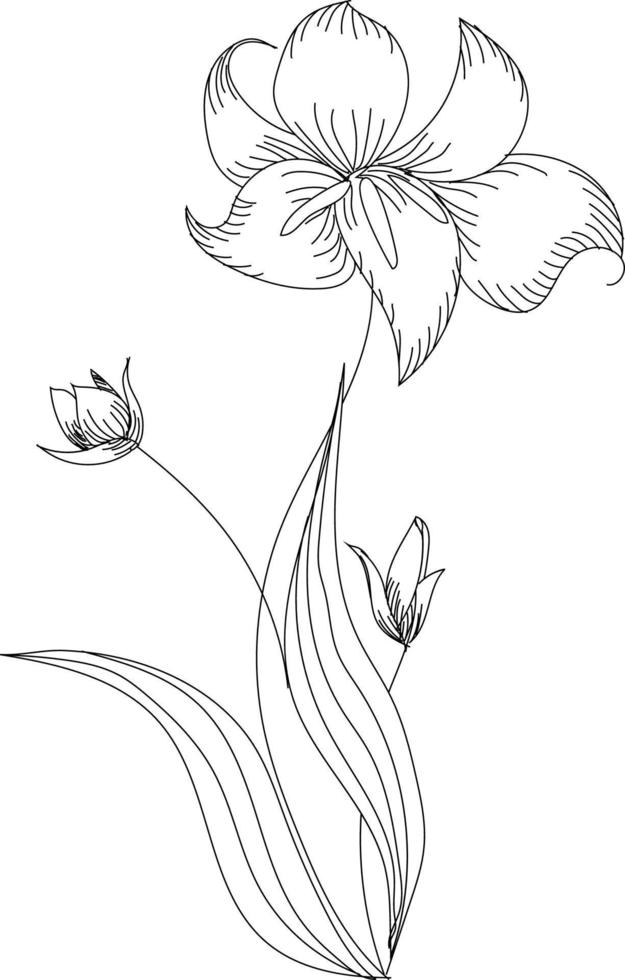This intricate pen and ink sketch depicts a stylized flower, predominantly resembling a lily with elements suggestive of tulips. Set in stark black and white, the composition features a flower with six triangular petals, radiating from a thin, singular stem that forms the primary axis of the drawing. Along this central stem, two additional blossoms emerge: a smaller flower with four petals on the left, and another budding flower with three petals on the right.

At the base of the central stem, two broad, curved leaves, marked with striped details, anchor the plant. The depiction of leaves and petals is highly stylized, with an artistic emphasis on symmetry and form. Notably, there is no background, allowing the flower to dominate the scene. The tallest flower, positioned at the top of the stem, is in full bloom, with pronounced central stamens enhancing its detailed appearance. The entire piece exudes a harmonious blend of botanical accuracy and creative interpretation, capturing both the delicacy and structure of the flowers in a minimalist yet expressive manner.